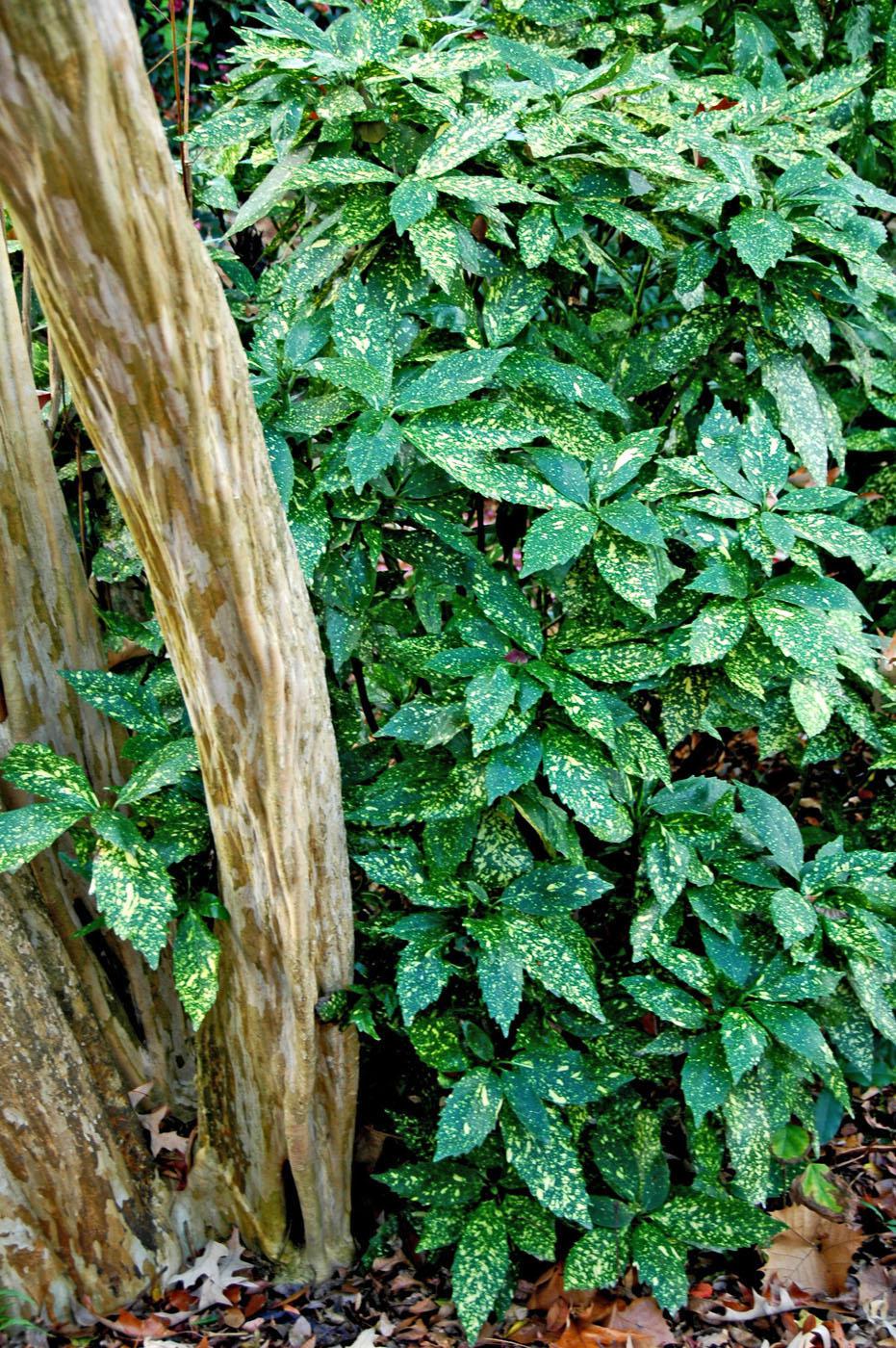The image showcases a vibrant outdoor scene with lush green leaves that are prominently speckled with yellow spots. The intensity and distribution of these yellow speckles suggest that the leaves might either belong to a specific plant species with naturally occurring spots or indicate potential issues like disease or insect damage. Positioned on the left side of the image is a brown-colored trunk or branch. Additionally, the scene includes several light brown tree stumps and a variety of dead leaves and wood on the ground, emphasizing the natural setting. The composition hints at a cyclical pattern in the leaves, arranged in clusters of four, contributing to the detailed and lively portrayal of this plant life.